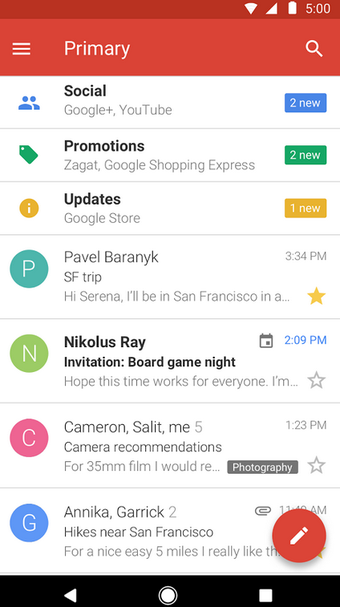The screenshot displays a phone's interface with a red status bar at the top that includes Wi-Fi and battery icons, along with the time showing as 5:00. Below the red bar, there's a lighter red section featuring a three-bar menu icon on the left, labeled "Primary," and a search icon on the right.

In the content area, there are seven distinct lines, each accompanied by an icon or emblem on the left side. The first three lines are in bold print with additional text in lighter font. The fourth and fifth lines also include lighter print text, while the sixth and seventh lines are entirely in lighter font. Each of the top three lines includes a different colored rectangle on the right side: blue for the first, green for the second, and yellow for the third. The fourth line is marked by a yellow star icon, while the fifth and sixth lines each have a hollow star icon, although the visibility of the fifth line is partially obstructed by a floating circular button with a pencil icon at the bottom right of the screen.

The bottom of the screen features a black navigation bar typical of an Android device, containing the "go back" button, a circle home button, and a square for recent apps, indicating an Android operating system. The exact application in use is unspecified.